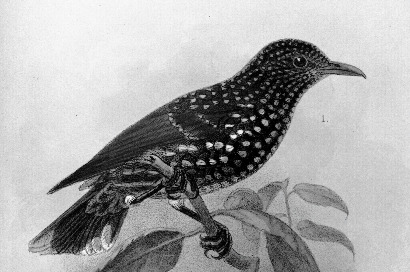This black and white image appears to be an intricate pen and ink drawing in the style of John James Audubon. It depicts a dark-colored bird, possibly a grackle, perched sideways on a thin branch. The bird is elaborately detailed, covered in pearlescent-like, silver or white specks that adorn its head, chest, back, and wings. Its beak is closed, and its sharp claws grasp the branch firmly. The tail is predominantly black with subtle white accents on the top edges. The branch, which extends directly towards the viewer, features several leaves, also rendered in black and white, making it impossible to distinguish the species without color. The background is a plain, soft white with subtle gray shading, providing a stark contrast that accentuates the crisp, meticulous details of the bird and the branch. A numeral "1." appears in the corner, but no additional text identifies the bird.